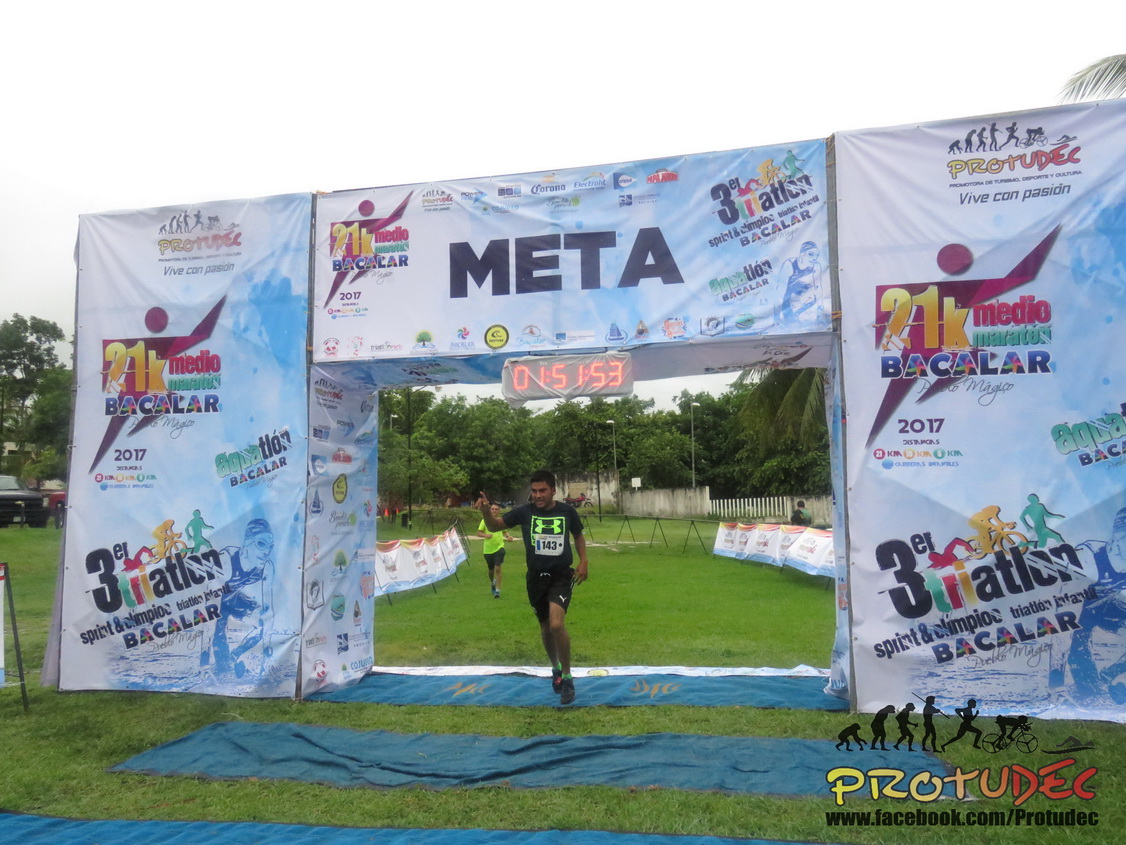In this detailed image of an outdoor summer race, the scene is set against a lush green grassy field, framed by a backdrop of numerous trees. The focal point is a large, boxy, built-out finish line structure adorned with various sponsor logos, prominently featuring "Meta" in dark letters at the top. Below the logos, an LED clock displays the time "1:51:53." 

A runner, dressed in a black shirt with a lime green Under Armour emblem, black shorts, and black shoes, is in the act of crossing the finish line. He is positioned under the top part of the structure, passing through a cutout section near a blue tarp that marks the finish. 

Another runner can be seen in the distance, roughly 20 yards away, wearing a bright green or yellow shirt and black shorts, also nearing the finish line. The race appears to be a triathlon, possibly organized by Produtech, as suggested by a logo in the bottom right-hand corner depicting a sequence of walking, running, and biking figures, alongside their Facebook page information. The overall color scheme of the finish line structure is blue and white, complemented by a myriad of other sponsor logos, indicating the event took place in 2017.